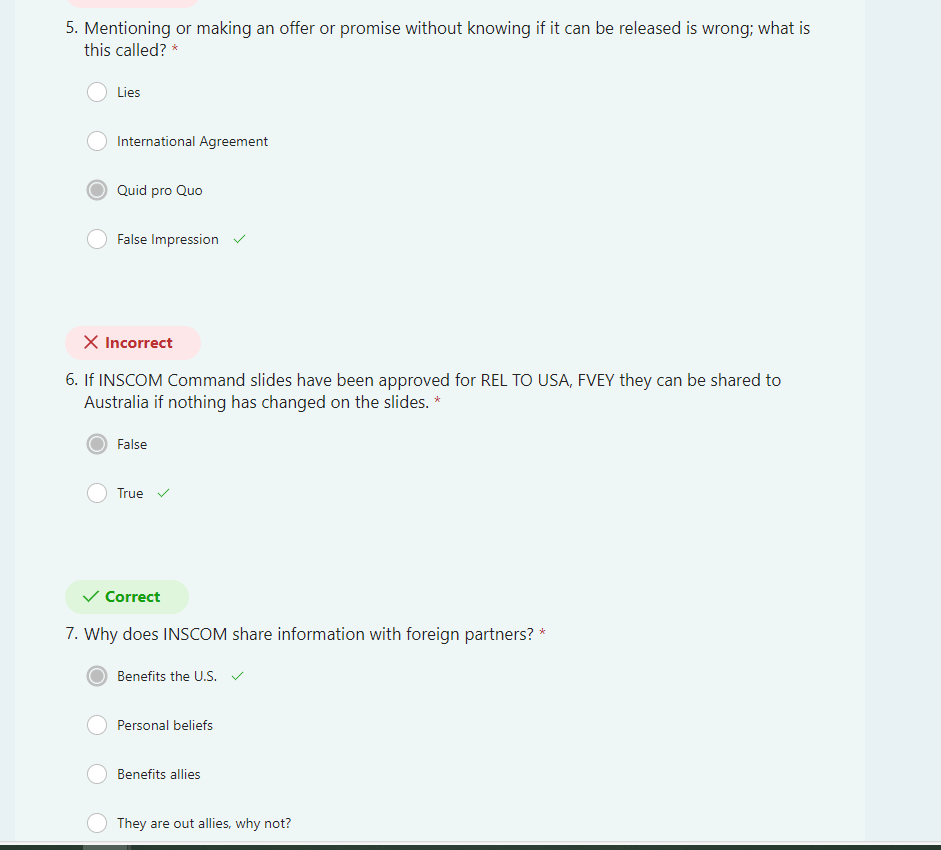This image features a gray background with a thinner, darker border in the same color, just a shade darker on the left side, and a thicker border on the right side. At the bottom of the image, there's a thin black line. At the top, the text reads "5," followed by a question: "Mentoring or making an offer or promise without knowing if it can be released is wrong. What is this called?" 

Four options are listed below this question with small circles next to each option:
1. Lies
2. International Agreement
3. Quid Pro Quo
4. False Impression

The person initially selected "Quid Pro Quo," which was incorrect. The correct answer, marked with a green checkmark, is "False Impression."

Following this, there's another question labeled "6" that reads: "If InScom command slides have been approved for route to USA, FVEY, they can be shared to Australia if nothing is changed on the slides." The options provided are "False" or "True." The individual chose "False," but the correct answer, indicated by a green checkmark, is "True."

The third question discusses the reason for InScom sharing information with foreign partners, with the options:
1. Benefit of the US
2. Personal Beliefs
3. Benefit Allies
4. They are allies, why not.

The selected answer was "Benefit of the US," which was correct and marked appropriately.